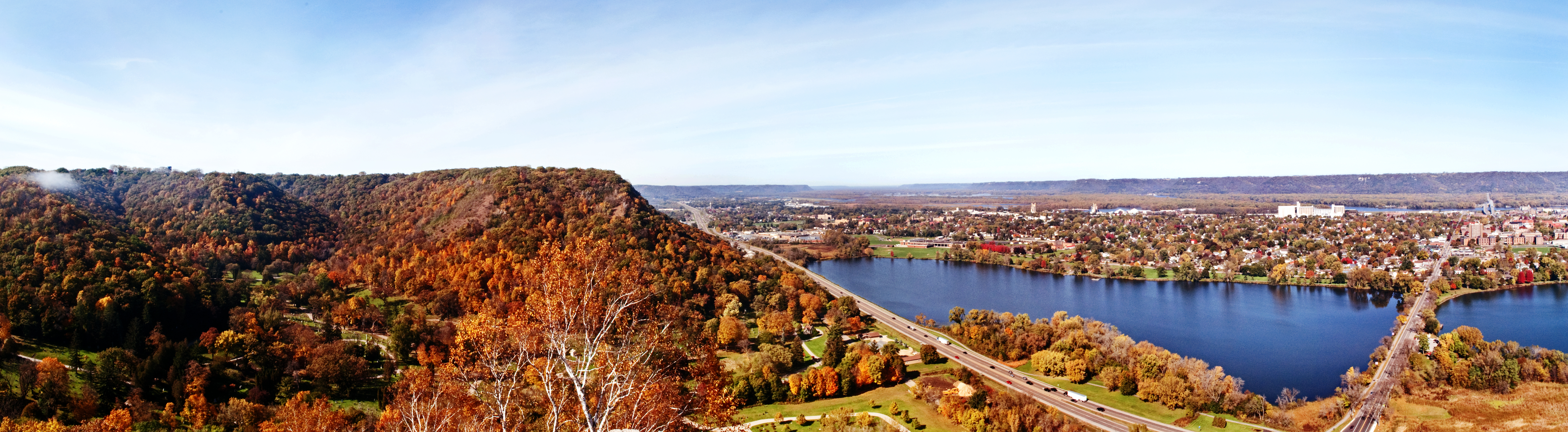This panoramic photograph captures a vibrant autumn landscape marked by a multitude of fall colors. On the left side, a hillside is draped in trees showcasing a palette of oranges, reds, browns, and yellows, typical of mid-fall. Interspersed among these are patches of evergreen trees, providing a contrast with their persistent greenery. Below the hillside, a road can be seen with cars navigating its path. 

As the scene extends to the right, a serene, expansive lake with deep blue water dominates the view. A prominent bridge spans the lake, connecting to the other side where a small town is nestled. The town is replete with dozens of buildings, interspersed among clusters of trees, and appears relatively compact with a mix of urban and rural elements. 

Further in the background, more water and hilly terrain stretch into the distance, creating a layered depth to the landscape. The sky above is a clear blue adorned with soft white clouds, rounding off this scenic vista of autumnal beauty and serene natural elements.